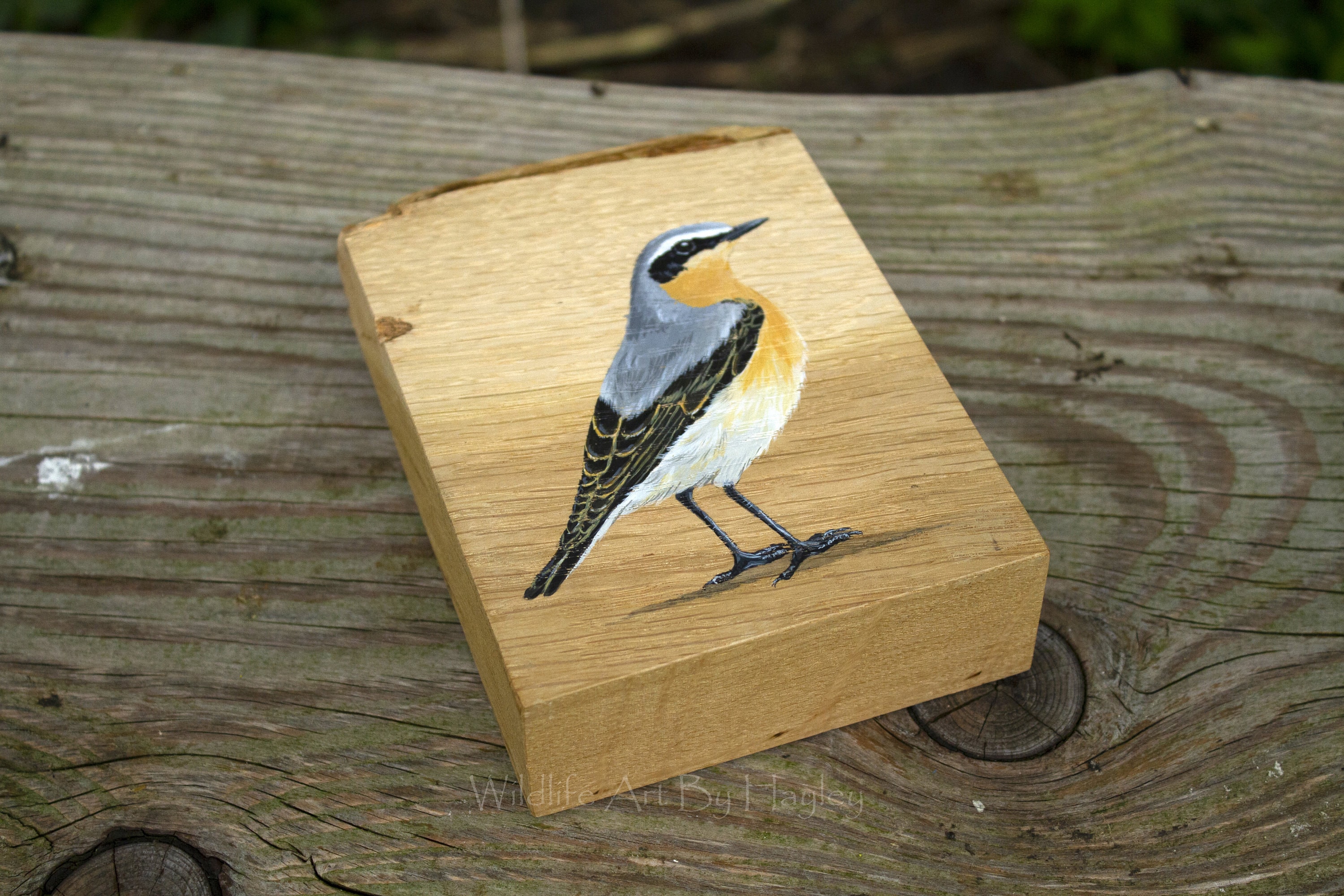The image showcases a painting of a small bird on a light brown, natural woodblock, which appears to be freshly cut and has a mostly straight edge with a noticeable nick on the left-hand side. The woodblock itself seems somewhat unfinished and jagged on the top. The bird in the painting features a light gray back and head, a distinct black mask that extends to its beak, which is also black, black wings with golden accents, and short black legs. Its chest is gold, transitioning to a white stomach. This woodblock rests on a weathered, gray plank of wood that resembles an outdoor deck, showing signs of age and exposure to the elements, possibly including what looks like bird droppings on the left-hand side. The contrast between the fresh woodblock and the aged plank emphasizes the rustic, natural aesthetic of the scene.